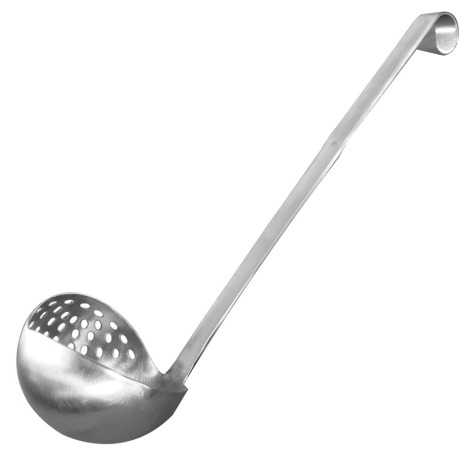The image depicts a unique silver soup ladle set against a plain white background. The ladle has a long, slender handle that curves inward at the top to form a round hook. The scooping section of the ladle is unconventional, as it is divided into two functional parts: one half is a solid bowl, and the other half features numerous small perforations, acting as a strainer. This design allows for the easy draining of liquids while scooping. The image is free of any text or additional elements, focusing solely on the distinctive, dual-sided ladle with one solid and one perforated section. The ladle appears slightly tilted, with the handle sloping upwards towards the top right corner of the image.